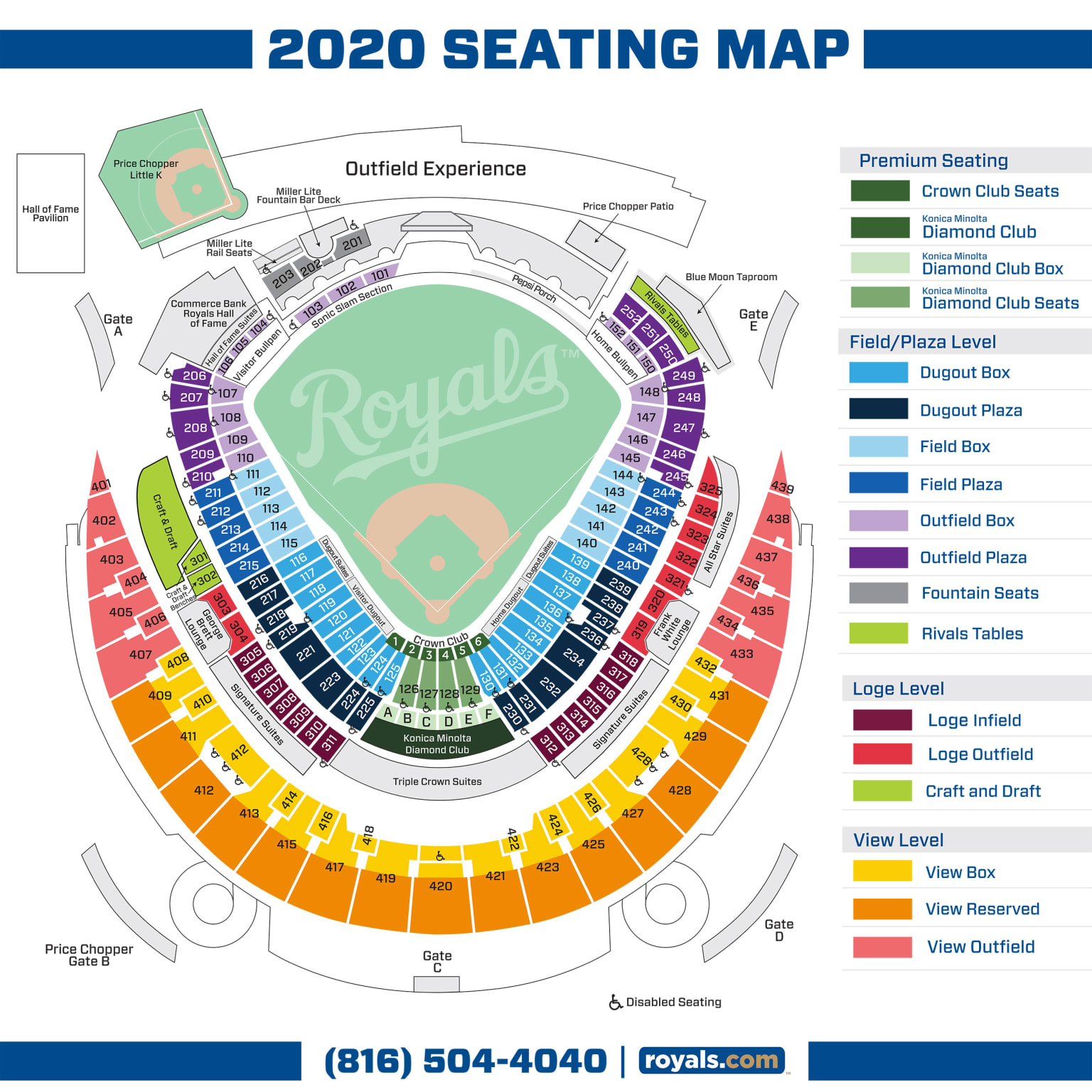This image showcases a color-coded seating map of a baseball arena, specifically designed for the year 2020. At the top of the image, the title "2020 Seating Map" is prominently displayed in blue, flanked by blue bars on either side for emphasis. The arena's seating sections are meticulously color-coded to indicate various seating tiers and areas. The baseball field at the center prominently features the word "Royals" in a stylized baseball script font. 

On the right side of the image, a detailed sidebar explains the color-coding system. It categorizes the seating options, starting with "Premium Seating" at the top. The list includes Crown Club seats, Diamond Club seats, Diamond Club boxes, Diamond Club seats, Field Plaza level seats, Dugout boxes, Dugout plaza seats, Field boxes, Field plaza seats, Outfield boxes, and Outfield plaza seats. Each category is represented by different colors, including shades of green, blue, and purple, providing a clear visual guide for prospective attendees.